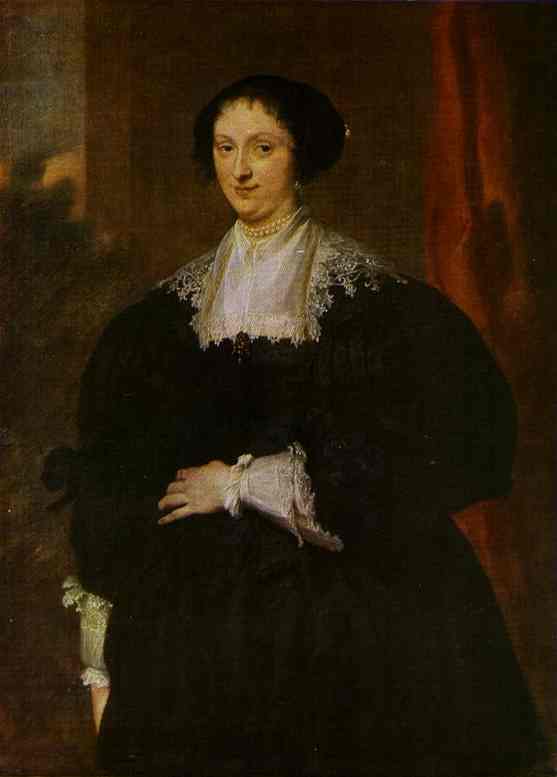This highly detailed portrait from the 1800s features a woman with fair white skin and short, rounded black curly hair that frames her face and covers her ears. She has brown eyes and a slight smile. The woman is elegantly dressed in a heavy, dark brown or black dress adorned with intricate lace detailing and silk around the neckline and sleeves. White lace also trims the dress's cuffs at her wrists.

Around her neck, she wears a delicate scarf, primarily white lace with hints of brown and gray, complemented by a double strand of pearls. Her left hand is placed over her stomach with fingers open, while her right arm hangs down by her side. Behind her, the backdrop includes a red-orange curtain on the right and a mix of dark green and gray shades on the left, suggesting a rich, yet understated setting typical of portraits from the era.

The overall composition and subtle details hint at her high social standing, perhaps suggesting she is either a member of a wealthy family or affiliated with a church.